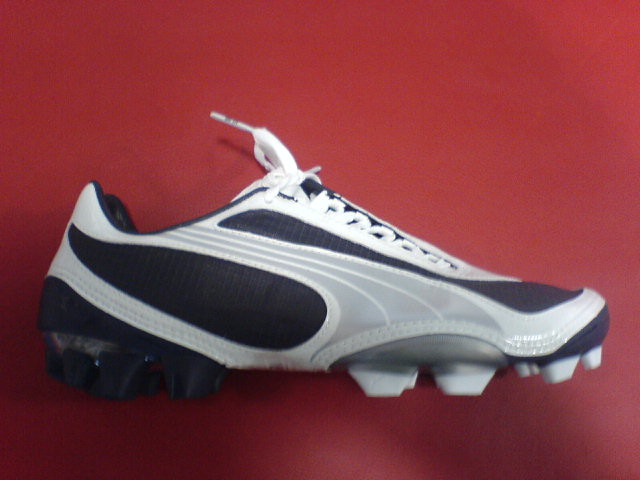The image showcases a close-up view of a cleat, possibly a soccer or baseball cleat, set against a gradient red background. The red background transitions from a lighter shade at the top to deeper shadows casting a dark, almost black hue in the bottom left and right corners. The shoe itself features a straightforward design, primarily black, white, and gray, with details suggesting both colors mentioned. It is adorned with white shoelaces. The cleat's bottom displays a series of spikes; the front spikes are white, while the back spikes near the heel are black. The shoe is oriented towards the right side, revealing gray stripes running lengthwise and black areas both at the heel and the front of the shoe. The clean and minimalist aesthetic of the cleat stands out prominently against the vivid red background.